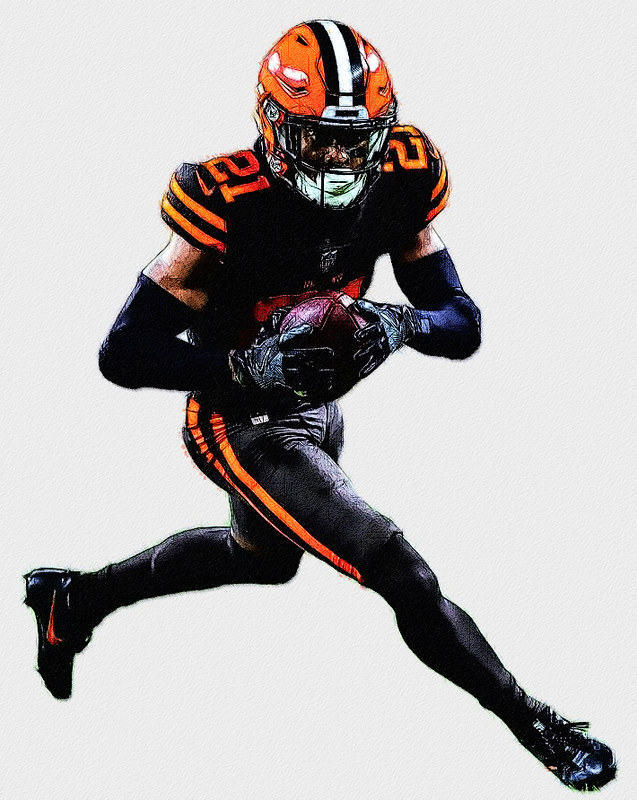This is a digitally rendered image of a football player set against a white background. The player, a black man, is depicted in motion, running with a football securely in his grasp. He is dressed in a striking black jersey adorned with orange accents, including orange lines on the sleeves and the number 21 printed prominently in orange on the shoulders. The jersey features the Nike logo above the sleeve lines. He also sports black gloves, black shorts with orange stripes on the sides, black leggings, and black boots with an orange Nike logo. An orange helmet with a white and black design stripe down the middle and a face mask completes his gear, adding to his dynamic and intense appearance. The image appears to be a drawing or heavily filtered, contributing to its distinctive and stylized look.